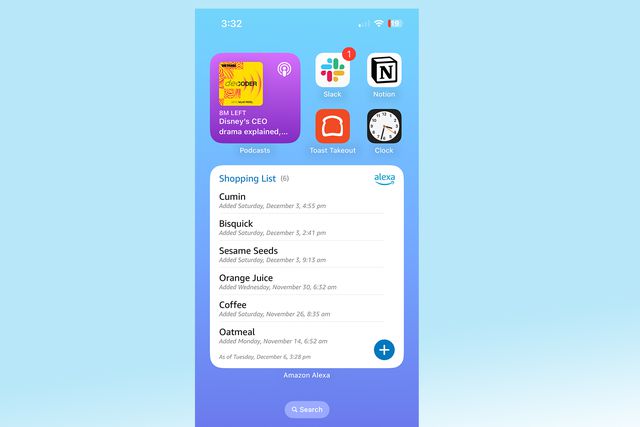This image, captured on a smartphone, displays a detailed shopping list. The phone screen is framed by a wide, light teal background, with the phone itself situated centrally. The phone's interface features a deeper periwinkle backdrop. At the top of the screen, the exact time is displayed as 3:32, alongside several status icons including signal bars, Wi-Fi, and a low battery indicator with a red strip. An advertisement headline reading "Disney CEO Drama Explained" with a note on time remaining ("8 minutes left") also appears.

Four app icons are visible at the screen's top left—Slack, Norton, Toast Takeout, and a clock icon. Below these icons, the title "Shopping List" appears in blue with a number six in parentheses, indicating the list's six items. To the right of the title, "Alexa" is noted. The shopping list consists of the following items: Cumin, Bisquick, Sesame Seeds, Orange Juice, Coffee, and Oatmeal. At the bottom of the list is a plus button for adding more items.